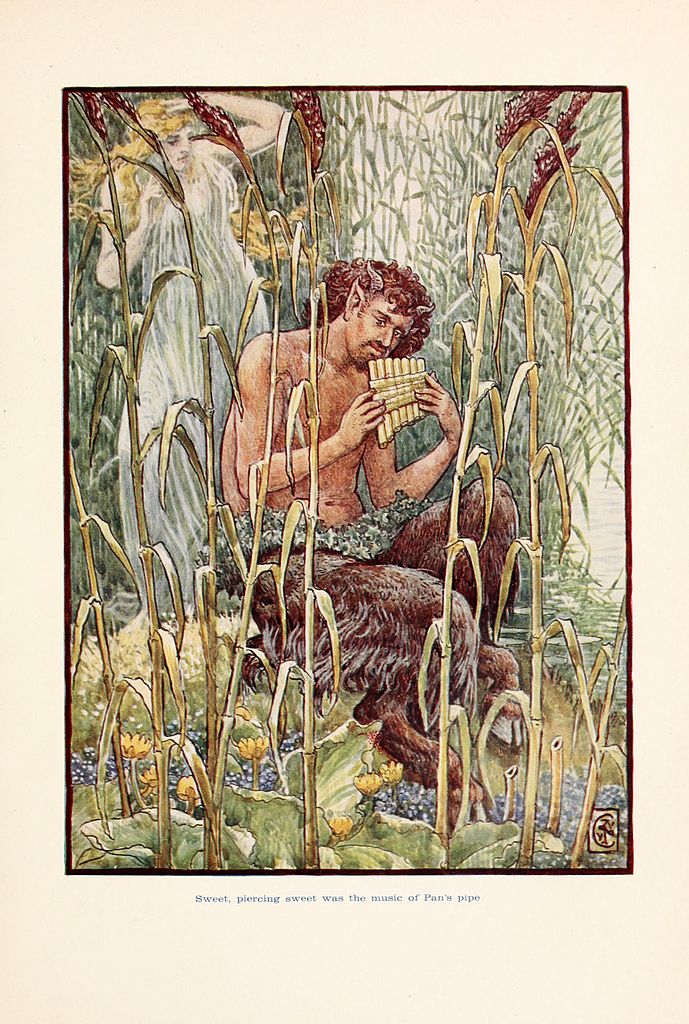The image is a tall, rectangular painting bordered by a dark reddish-black color against a beige background. Below the painting, a small blue font reads, "Sweet, piercing sweet was the music of Pan's pipe." The painting depicts Pan, a mythological creature with the torso of a man and the legs of an animal, complete with horns, pointed ears, cloven hooves, and curly hair. He is sitting by a light blue body of water overgrown with light green reeds, and he is playing his signature pipe. Pan's nude torso is prominently centered in the painting. Behind him stands a woman with pale skin and long, flowing blonde hair, wearing a diaphanous white gown that catches the breeze. She holds her hands up in surprise. The scene is colored in muted tones, predominantly featuring greens, browns, golds, and the natural hues of Pan's skin. The water and surrounding foliage add layers of depth to the composition.